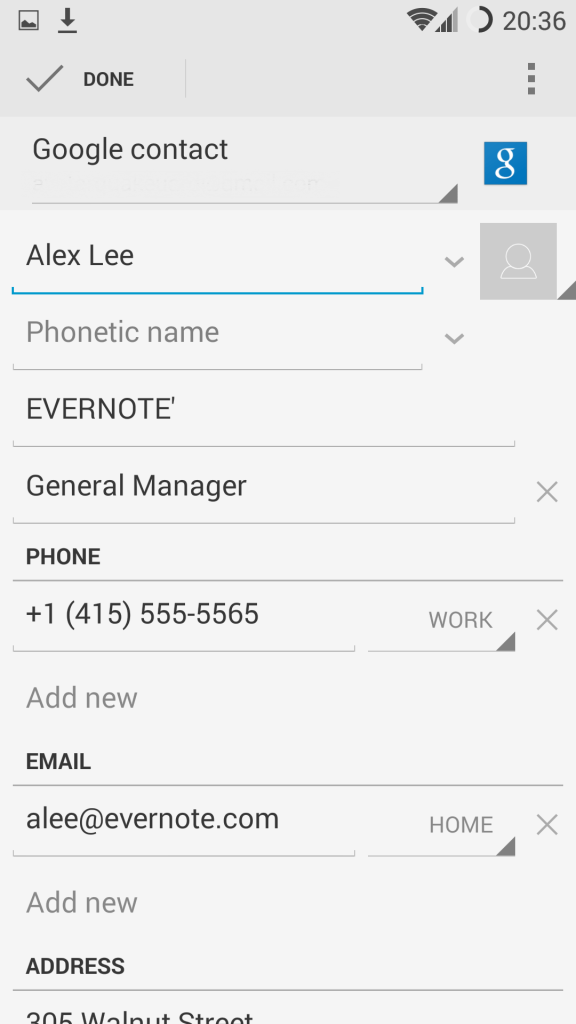The image is a screenshot of an Android device displaying the contact-saving interface. The user is adding a new contact named Alex Lee. Various fields are filled out as follows: the phonetic name is left blank, and a note stating "Evernote" is included. Alex Lee’s position is listed as "General Manager." The contact information includes a phone number, +1 (415) 555-5565, and an email address, a.lee@evernote.com. The partial address shown is 305 Walnut Street.

In the interface, the top-left corner features a small icon, indicating that the screenshot was taken. Adjacent to this is a downward arrow pointing to a line, symbolizing the download option. The top-right corner reveals that the device is connected to Wi-Fi with two bars of data coverage. The time displayed is 8:36 PM. Additionally, a unique icon—a circle half white and half black—is visible, though its function is unclear.